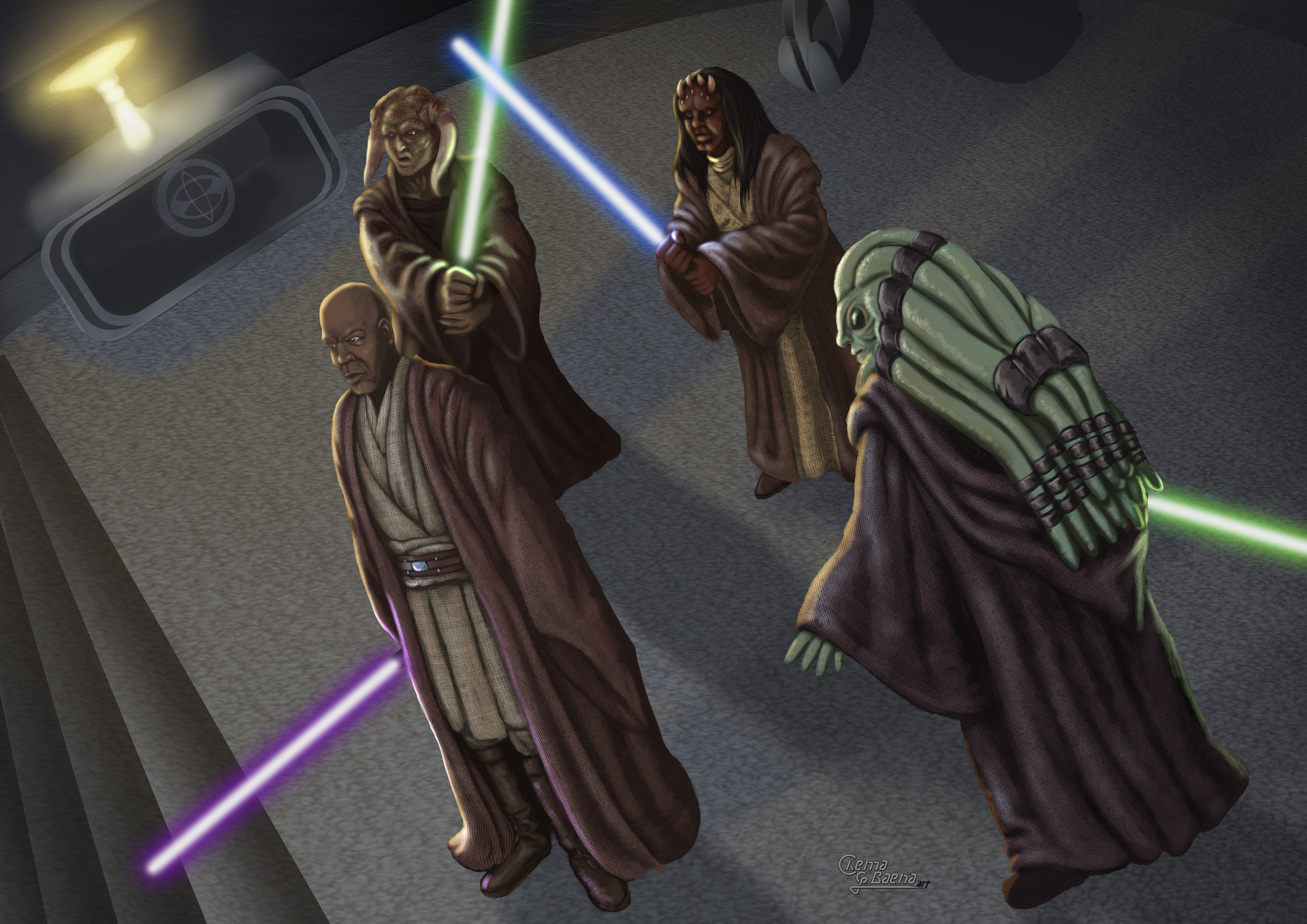The image depicts a scene reminiscent of a Star Wars-themed video game or cartoon with four Jedi characters, each holding lightsabers and dressed in dark robes. On the leftmost side stands a bald Jedi, donned in a tan off-white garb and a brown-purple robe, holding a purple lightsaber pointed towards his waist. Directly behind him is a Jedi with horns braided together as hair, clad in a brown and gray robe, holding a green lightsaber with both fists. To this character's right and somewhat centrally positioned is a female Jedi, identifiable by her long hair and four small horns on her forehead. She wears a tan and brown garb with a brown robe and crosses her blue lightsaber with the green one next to her. On the far right is a Jedi with long, green, snake-like hair, a green face, large black eyes, and green fingers protruding from the robe. This character holds a green lightsaber to his side. The group is assembled on a dark gray platform with several stairs leading up to it in the lower left corner, and behind them is a glowing yellow pedestal on a rectangular table with a circular insignia.